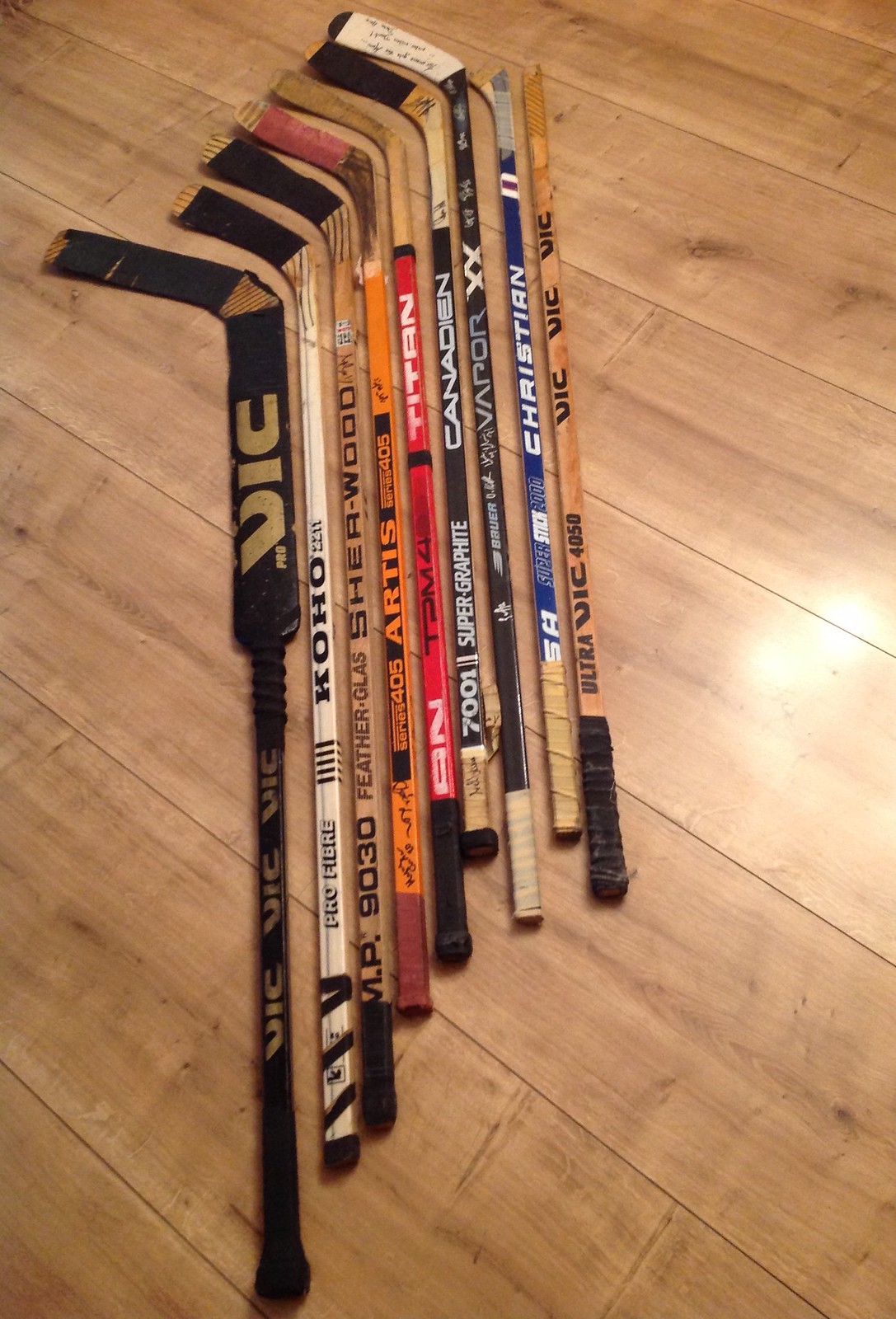The image features a collection of nine hockey sticks, side by side, strategically arranged on a light brown hardwood floor with visible wooden grain and knots. The picture, taken directly from above in a portrait orientation, showcases the sticks running vertically from top to bottom. There is an overhead light source casting varying shades of brightness on the floor. Among the nine sticks, two on the ends are broken, missing the bottom parts where the puck is struck. The longest and thickest stick, primarily black, is on the far left, while the others vary in size and color. Each stick displays different brand names and colors, such as Ultra Vic 4050 Vic, SA Super Stick Rude Christian, Bauer Vapor XX, 7001 Super Graffiti Canadian, T2 M4 Titan (in red), Series 405 Artist Series 405 (in orange), MP9030 Feather Glass Sherwood, Pro Fiber Coho, and Vic repeated multiple times. Most sticks have white tape wrapped around their handles, with one featuring red tape. The diverse assortment of sticks, detailed with various brands and colors, highlights their distinct styles against the wooden floor backdrop.